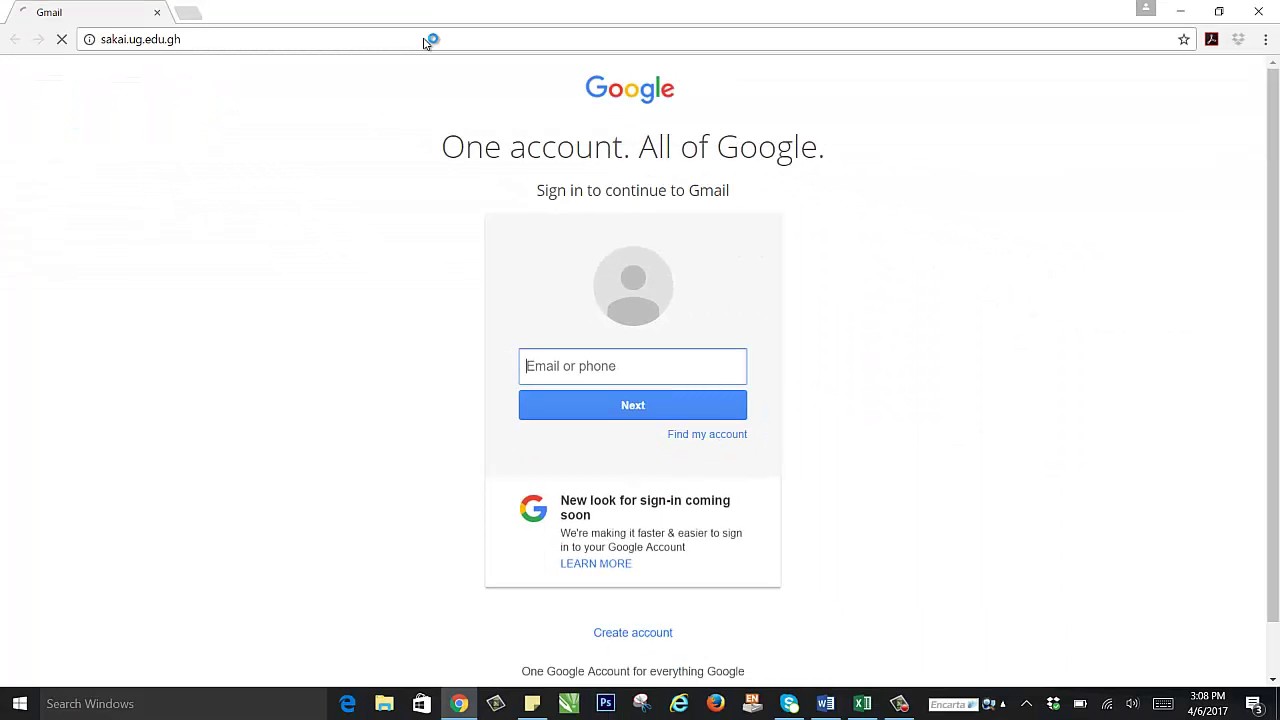This image displays the Google sign-in page on a PC. At the top, the Google logo is prominently featured with the tagline "One account. All of Google." Below this, there is a prompt to enter either your email address or phone number, followed by a blue "Next" button. If you have trouble accessing your account, there's a "Find my account" link at the bottom. A banner announces a new look for signing in, along with a "Create account" option in blue. The desktop's black taskbar is visible at the bottom of the screen, displaying icons for various applications, the weather, and the time. Above the taskbar, there's a reminder that "One Google Account for everything" emphasizes the unified nature of Google's services across devices. This visual captures the initial step for users to sign into their Google account on a computer, ensuring that their data and services are synchronized seamlessly across devices.